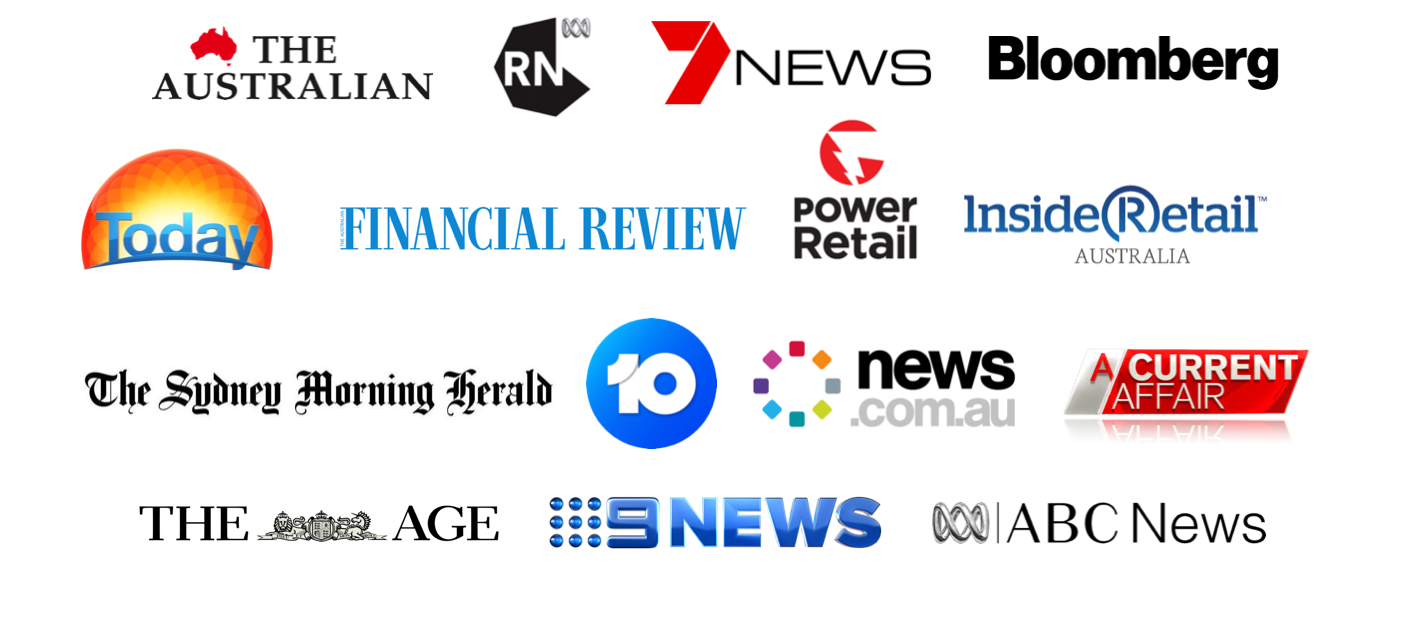This image features an array of various logos meticulously arranged in rows. Here’s a detailed breakdown:

- **Top Row (Left to Right)**:
  - The first logo features the word "Australian" in black text. To the upper left of the text, there is a red silhouette of the island of Australia.
  - Next, the "RN" logo appears, with the letters "RN" in white against a black semi-circular background.
  - The following emblem is for "Channel 7 News." The number "7" is in red, resembling two interlocking pieces of paper, while the word "News" is in black.
  - At the far right, the logo "Bloomberg" is displayed in bold black font.

- **Second Row (Left to Right)**:
  - The word "Today" is written in blue, set against a sun-like background.
  - "Financial Review" is written in blue text.
  - "Power Retail" is next, with a red circle and a lightning bolt symbol above it.
  - To the right, "Inside Retail Australia" is displayed, with a noteworthy design where the "R" in "Retail" is encircled.

- **Third Row (Left to Right)**:
  - The logo "The Sydney Morning Herald" is partially covered up and appears as "The Sydney Morning Carol."
  - "10 News.com AU Current Affair" is shown next.

- **Last Row (Left to Right)**:
  - "The Age" logo appears, followed by "9 News," and lastly, "ABC News."

Each logo is distinctively colored and styled, representing various well-known news and media outlets.